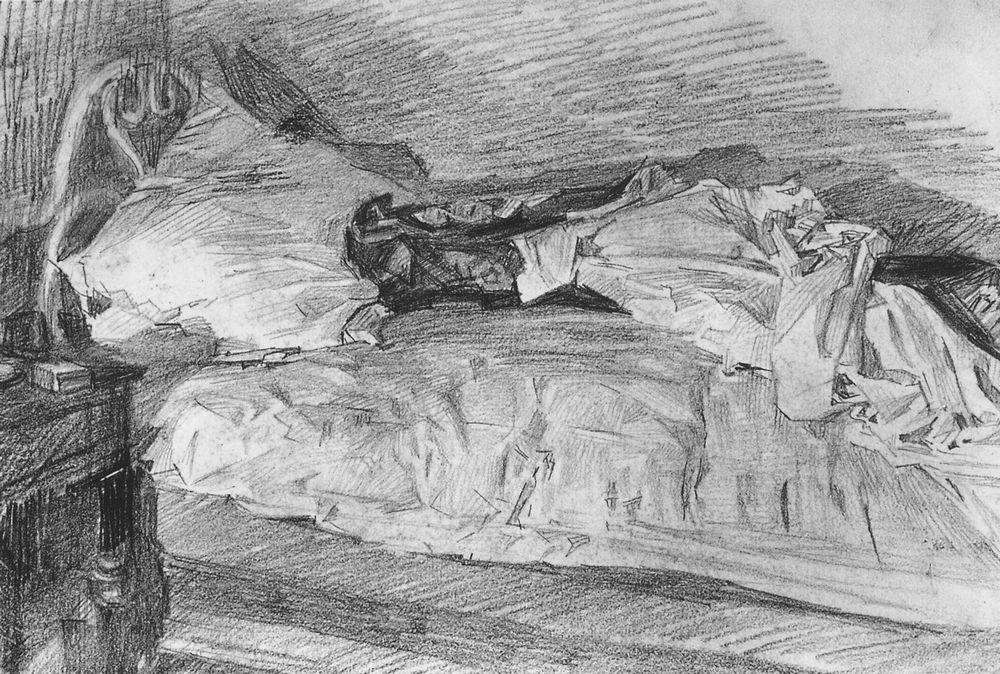This is a black and white pencil drawing, characterized by a fast and loose style, depicting a messy, unmade bed with detailed shading that gives the room depth and texture. The bed, complete with an elaborate headboard, boasts a large, dark-colored blanket partially thrown to the side, revealing white sheets beneath and a single pillow. Emerging from the rumpled sheets is a dark figure with a barely discernible face, positioned on its side, wearing dark clothing and covered by a white blanket, blending ambiguously into the bed, evoking a sense of abstraction. To the left of the bed stands a dark nightstand with matches atop, hinting at an older setting. The walls and floor display subtle shadows, adding to the drawing's atmospheric depth and intrigue.